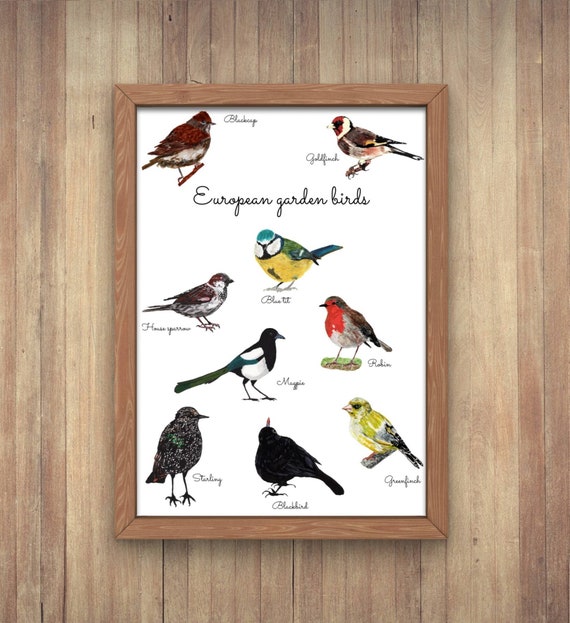The image is a detailed photograph of a brown wooden picture frame hanging on or placed against a light to medium-brown wooden panel wall made of narrow planks. The frame encloses an illustration titled "European Garden Birds" in cursive script. This illustration features nine different birds, each accompanied by a hard-to-read label in small print.

In the top left corner, there is a bird with a dark brown body and white breast. The top right corner features a smaller bird with a rust-colored head, white stripe, brown and black feathers, and a gray breast with red smudges near the tail. Beneath the title in the center is a brightly colored bird with a blue head, black and white mask, yellow body, and green back.

To the left of the colorful bird is another small brown and white bird, while to the right is a European robin with a red breast, brown upper parts, and white underparts. Below this robin is a larger magpie, displaying a black head, chest, back, and tail with some white on its stomach and side.

In the lower left corner is a starling with a black body interspersed with fine white dots, and to its right is an entirely black bird, potentially a blackbird, looking upward with its orange beak. Finally, in the bottom right corner is a greenfinch, characterized by its yellow and green body, and black-tipped wings.